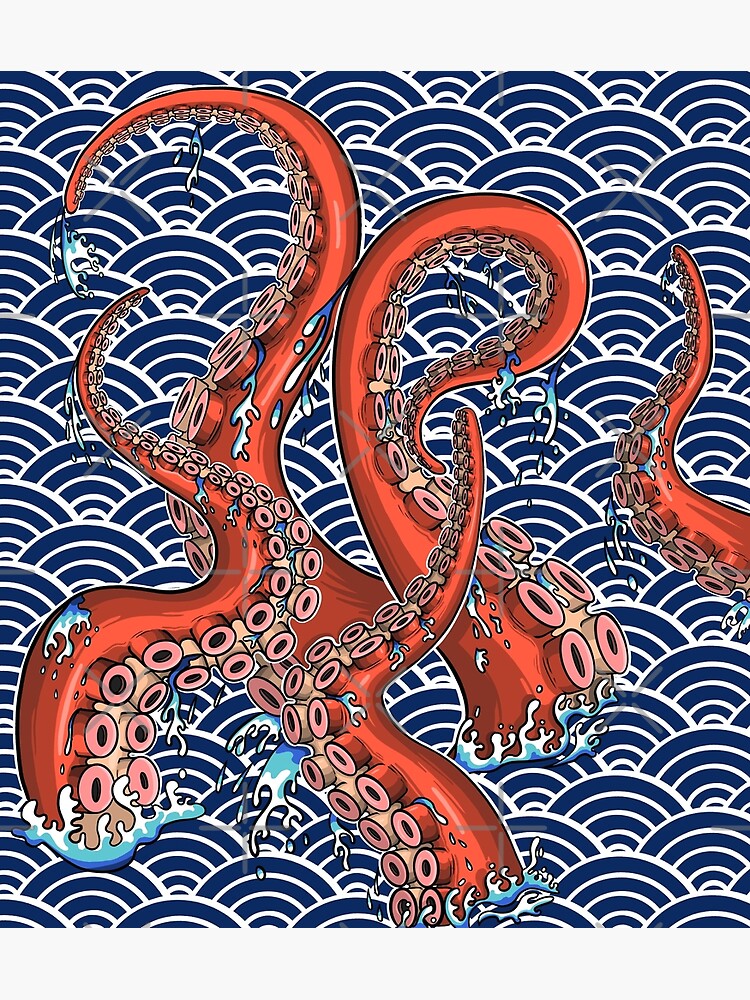The image seems inspired by Japanese folklore, depicting a kraken-like creature, possibly an octopus or squid, emerging from the ocean. The central elements are five tentacles in vivid shades of bright red and orange, marked with pink suction cups that vary in size, starting larger at the base and getting smaller towards the tips. The tentacles twist and curve in multiple S shapes, showcasing intricate, swirly designs and dotted with circular patterns. The ocean is represented abstractly with overlapping blue and dark blue semi-circles, highlighted by white lines that mimic the movement of water. Additional details include scattered water splashes and hints of fish caught among the tentacles, enhancing the dynamic and somewhat ominous nature of the scene. The artwork appears to be computer-generated, carrying a stylistic nod to Japanese cartoons or traditional art styles.